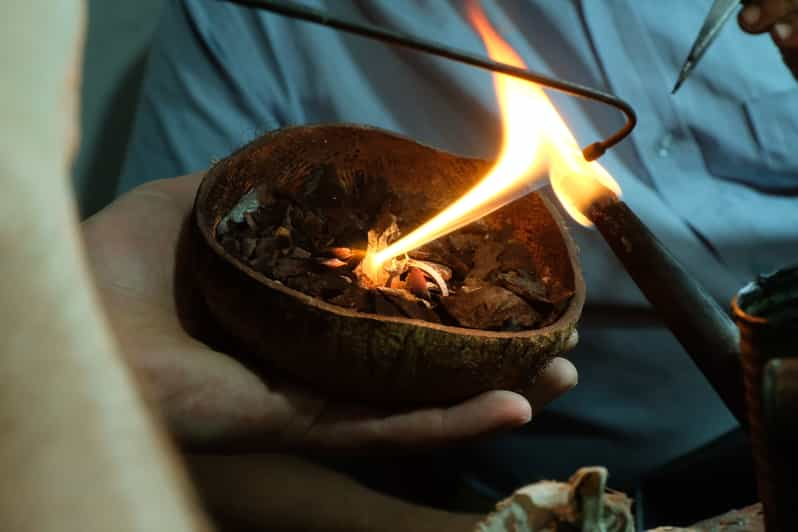The photograph is a close-up shot, wider than it is tall, centering on a hand holding a horizontally halved coconut shell, which appears ceramic or metal. Inside the shell are dried leaves or similar items. The hand belongs to a person whose arm extends from the left middle of the image. In the scene, two sources of flame are evident: a black torch from the bottom right and a thin metal prong from the top left, both directing yellow flames into the bowl. The intense fire is central, illuminating the medium blue button-up shirt and partially visible arm of another individual in the background. The setting reveals subtle, indistinct elements on the image periphery, adding to the focus on the dynamic interplay of fire and the contents of the coconut shell.